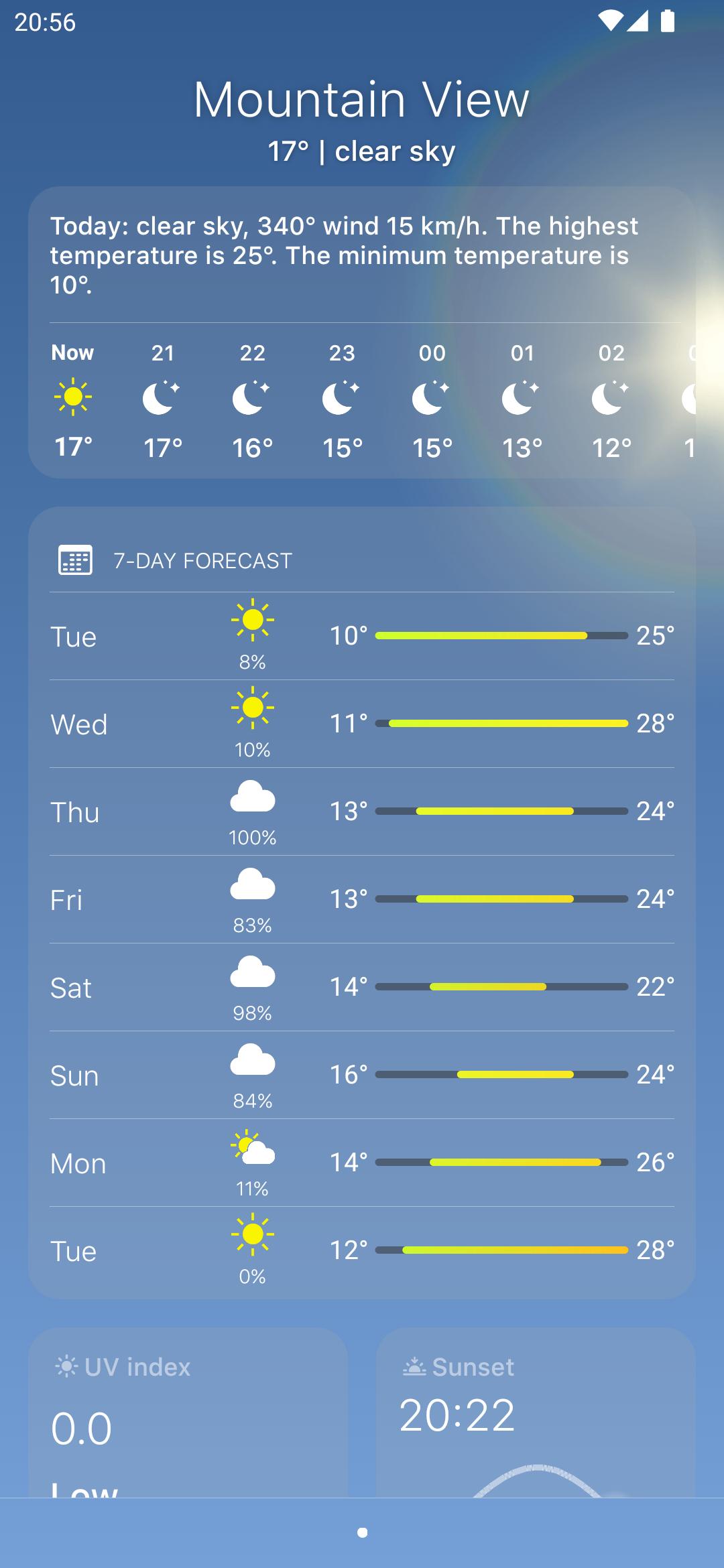**7-Day Weather Forecast with Detailed Conditions**

- **Today:** Clear skies with a light breeze from the northwest at 15 km/h. The highest temperature is expected to reach 25°C, while the minimum temperature will drop to 10°C. Currently, it is sunny with a temperature of 17-21°C, and clear visibility.

- **Evening Conditions:**
  - At 22:00, a half moon will be visible with a temperature of 16°C.
  - At 23:00, a half moon continues with a temperature of 15°C.
  - At 00:00 and 01:00, the half moon persists, and temperatures are 15°C and 13°C respectively.
  - By 02:00, the temperature will be around 12°C.

- **7-Day Forecast:**
  - **Tuesday:** Mostly sunny with temperatures ranging from 10°C to 25°C.
  - **Wednesday:** More sunshine with temperatures steady around 10°C.
  - **Thursday:** Clouds increasing with an overall 100% cloud cover and temperatures peaking at 24°C.
  - **Saturday:** Predominantly cloudy with a 98% cloud cover, temperatures ranging from 14°C to 22°C.
  - **Sunday:** Partly cloudy with an 84% chance of clouds, temperatures between 16°C to 24°C.
  - **Monday:** Mostly sunny with minimal cloud cover (11%), temperatures between 14°C and 26°C.
  - **Tuesday:** Clear skies with no cloud cover, temperatures will range from 12°C, and a high reading of 78°C (assumed to be a typographical error, likely meant to be 28°C), low UV index at 0.0.

- **Sunset:** The sun will set at 20:22 today.

The background of the forecast is a calming blue, and Monday is indicated by a small white dot on the weekly forecast chart. Thank you for following this week’s weather update.